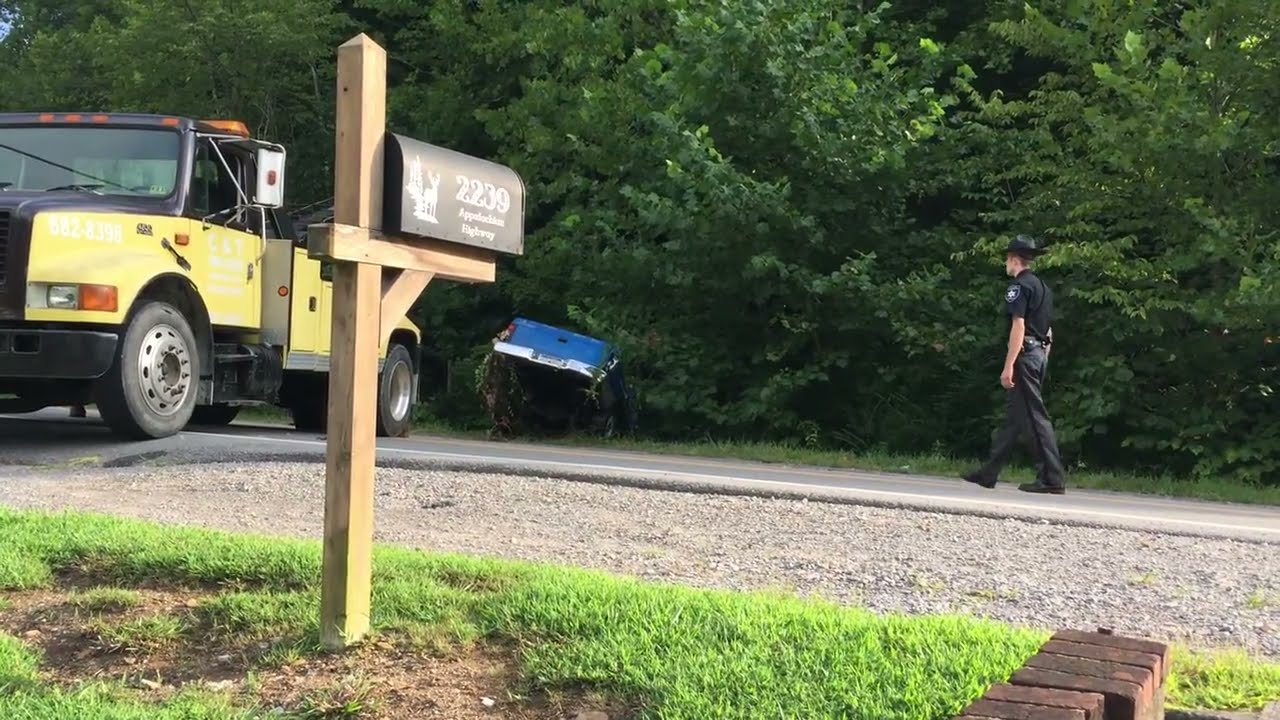The image depicts an accident scene set in an outdoor daytime setting. The backdrop features a long row of thick, bushy hedges or trees. In the foreground, a grassy yard hosts a black mailbox mounted on a wooden pole, marked with the numbers "2239" and adorned with an abstract white deer illustration. To the left side of the image, spanning the road, there's a modern yellow tow truck with black wheels, a black frame, and orange accents above the windshield, partially obscuring a blue vehicle. This blue vehicle is nosed down into a ditch along the tree line, with its tail end up in the air, suggesting it might be the rear of a pickup truck. Notably, the back bumper of this vehicle is entangled with roots and grassy debris. On the right side of the image, a Caucasian police officer dressed in a black uniform and hat, adorned with a badge, walks towards the tow truck, signifying the ongoing response to the accident.